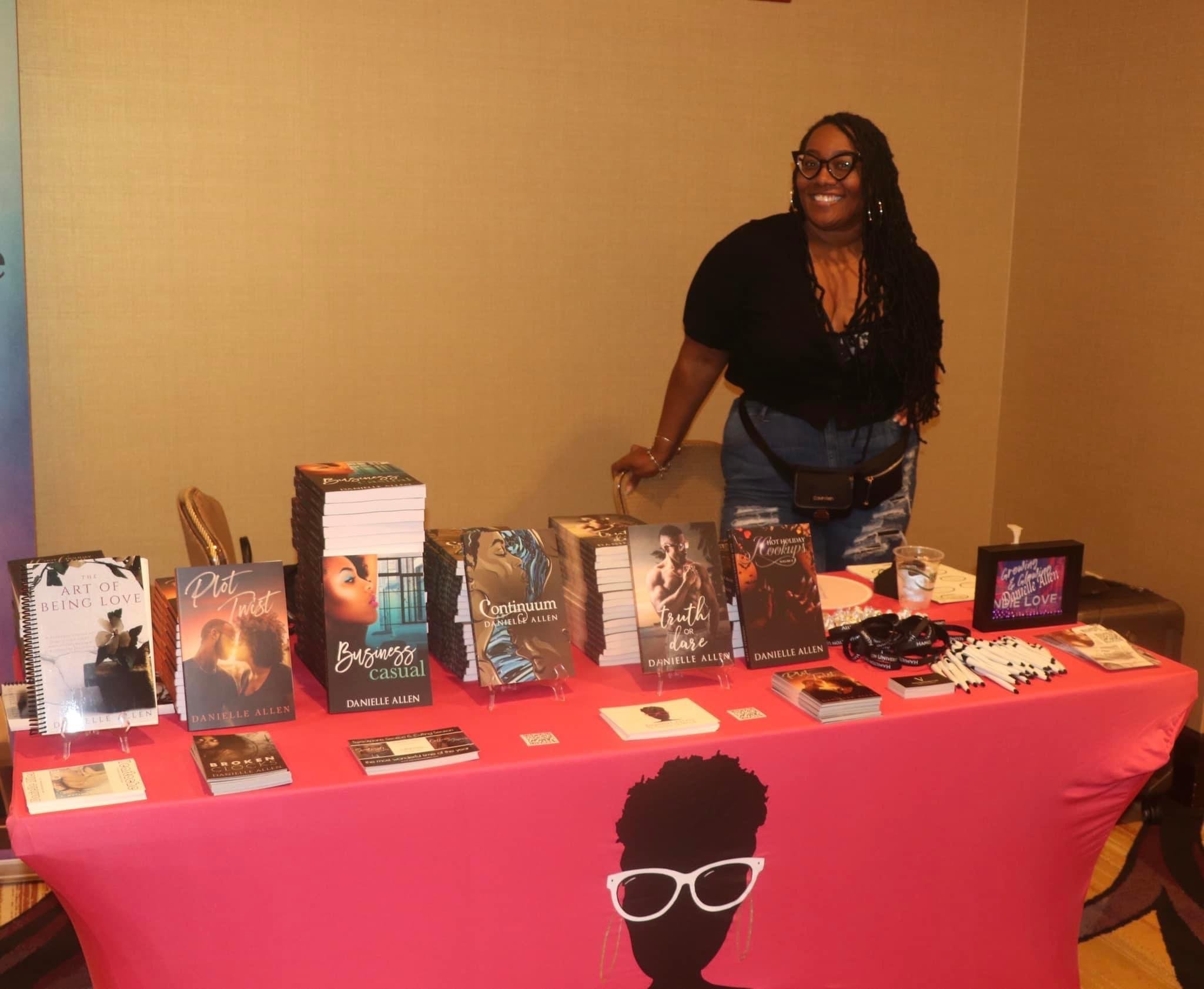The horizontal, landscape-oriented image depicts an African-American woman standing behind a red-draped table at a book show. The woman, presumed to be Danielle Allen, the author of the books displayed, is around 35 years old and smiles warmly at the camera. She wears long braided extensions, black glasses, and a black top, though her pants are not clearly visible. The table is adorned with a bright red tablecloth that features a graphic of a black woman wearing white glasses, mirroring the woman in the image. On top of the table, there's an array of romance books authored by Danielle Allen, including titles like "Art of Being Loved" and "Plot Twist," which features a photo of a couple kissing. Additionally, there's a pile of pencils and other items that might be giveaways, suggesting a book signing event. The entire scene is vividly captured in a style that accentuates the realistic and representational elements of the setting.